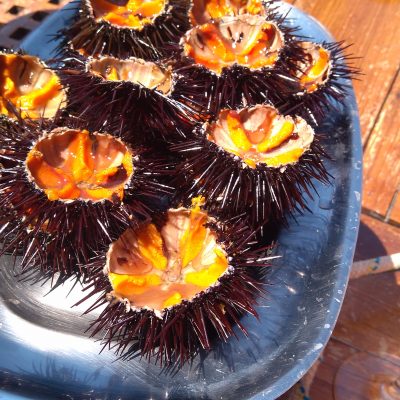The image depicts a painting of a blue, square-shaped platter with gently curved edges, holding nine sea urchin halves. These sea urchins are distinctive with their spiky, brownish-red outer shells, densely covered with hair-like spines. Each sea urchin has been cut open to reveal its interior, which showcases a smooth surface featuring a striking pinwheel design of pink and yellow hues. The platter itself rests on vertically aligned, bright brown, tan-colored wooden planks, giving it a rustic yet polished appearance. This close-up view highlights the intricate details of both the sea urchins and the contrasting wooden background, creating a vivid and textured composition.